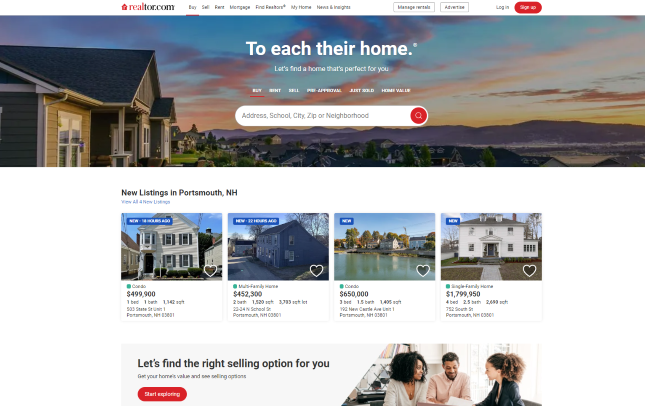The webpage features an array of detailed elements aimed at facilitating real estate activities. At the top, there is a logo with an image of a red house alongside the text "realtor.com," where "real" is highlighted in red, and the remaining text in black. The main navigation bar includes categories such as Buy, Sell, Rent, Mortgage, Big, Real Short, My Home, and News and Insights. Two buttons, labeled "Manage Rentals" and "Advertise," appear in a white box with a black or gray border, followed by "Login" and a red oval button with the white text "Sign Up."

Below the navigation bar, a picturesque image is prominently displayed. The foreground features a house surrounded by a community of homes, set against a backdrop of mountains under a sunset sky imbued with red and orange hues. The house on the far left corner is green with numerous windows and lush greenery around it.

Under this image, a white box highlights new listings in Pottsburg, NH. In blue text, it prompts users to "View all for new listings." Four property listings are detailed from left to right:

1. A condo priced at $499,900 with one bed, one bath, 1,342 square feet, and an address that is hard to discern.
2. A multifamily house listed at $405,300 featuring two baths, 1,520 square feet, and a lot size of 3,783 square feet, with a blurry address.
3. Another condo priced at $650,000 with three beds, 1.5 baths, and 1,405 square feet, including an address.
4. A single-family home priced at $799,950 offering four beds, 2.5 baths, and 2,683 square feet, with an address.

At the bottom of the listings, a section encourages users to "Find the right selling option for you, get your home's value, and see selling options." There is a red oval button with the call-to-action "Start Exploring." To the right of this section, an image depicts three people in an office setting with a white background: two women and a man in the middle, conversing and holding papers.